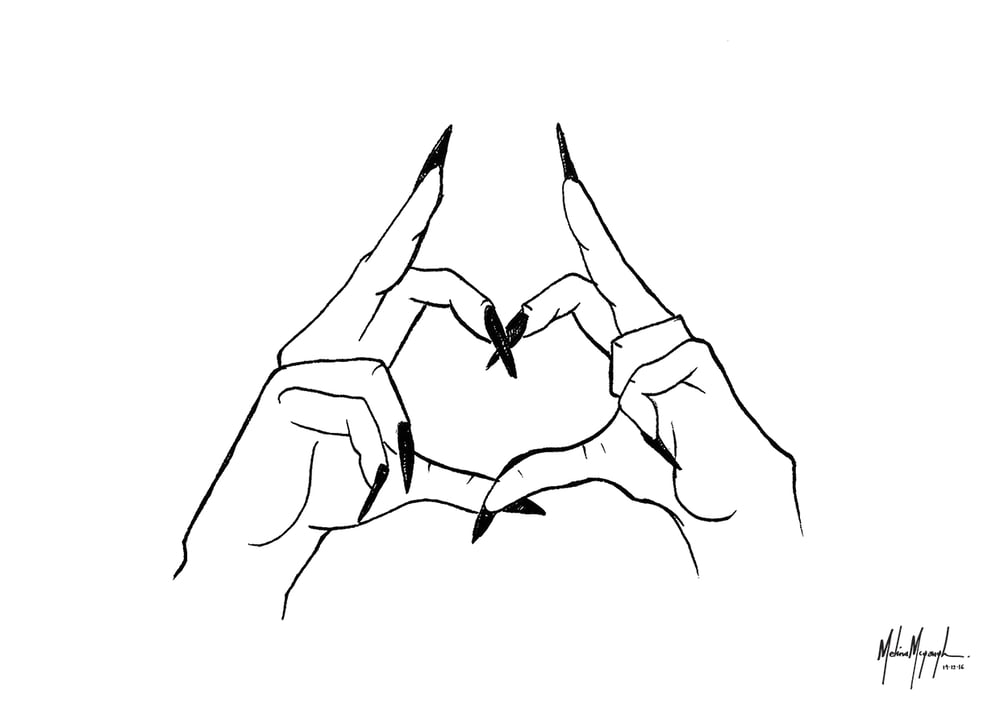This detailed black-and-white line drawing features two bony hands with extraordinarily long, black, talon-like fingernails. The hands are arranged to form an imperfect heart shape in the center of the image, with no border around it. The index fingers are curled down, creating the top curve of the heart, while their long, pointed black nails cross each other like an X. Both middle fingers point upwards at an angle and would intersect if imaginary lines were drawn along their length, although a small gap separates them. The ring and pinky fingers are bent inward toward the palms, with the left hand displaying both nails clearly, whereas the right hand only shows one visible nail as the other is hidden. The thumbs, extending across the middle, shape the bottom part of the heart without crossing each other, and their nails are prominently displayed. Below the hands, extending merely to the wrists, is an artist's signature located in the lower right corner. Although somewhat illegible, it features angular, straight-line lettering reminiscent of an electrocardiogram with up-and-down spikes.